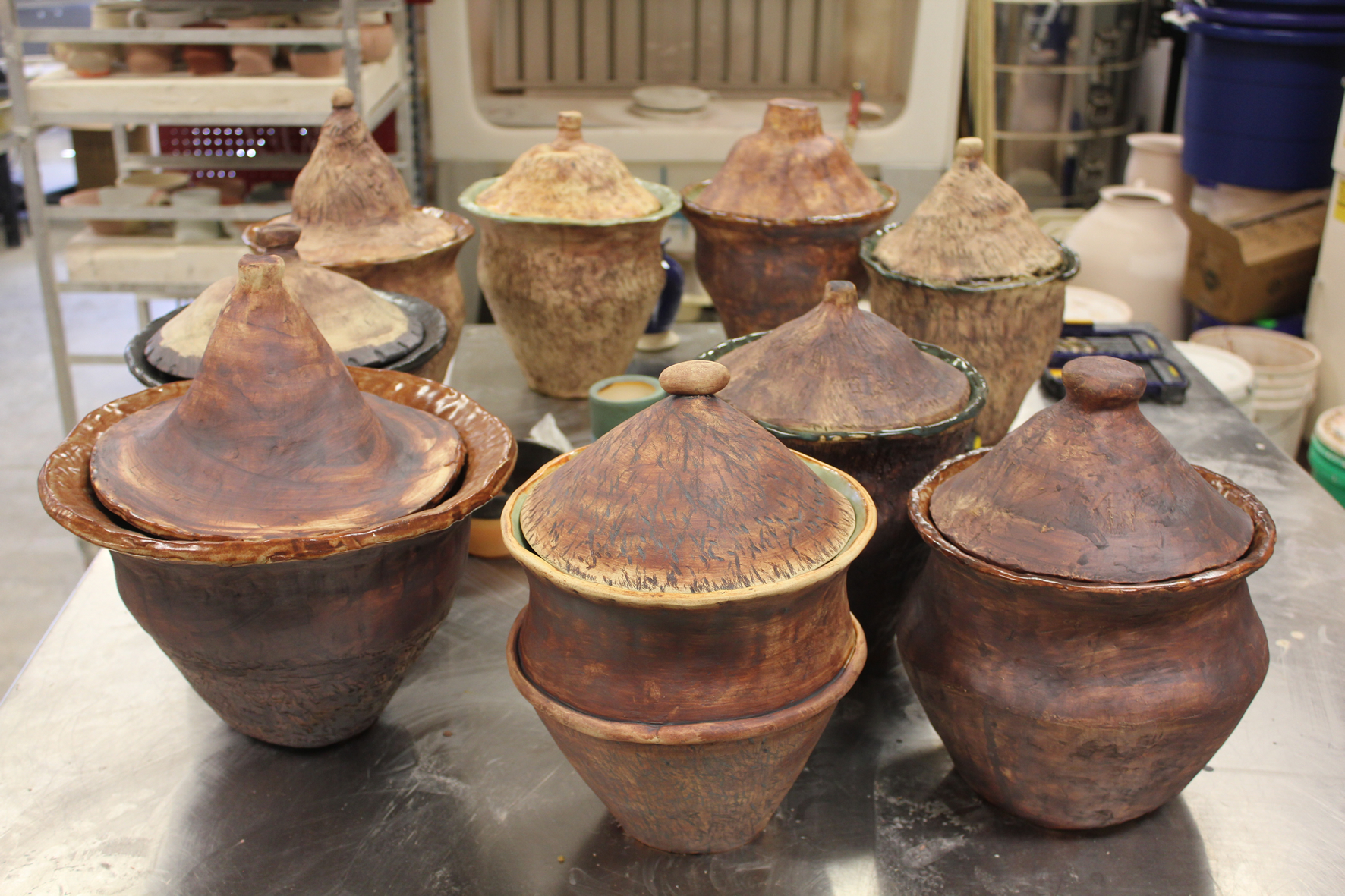The photograph showcases a diverse collection of sculpted clay pots, each characterized by its unique style and finish. All pots feature distinctive conical lids topped with small knobs, resembling containers that could hold anything from sundries to sundaes with cherries on top. The pots vary in color and glazing, set against a flat, scratched, and dirt-flecked metal surface, likely steel. This surface houses the pots arranged in slightly curvy rows: a back row of three or four, a middle row of two, and a front row of three. In the top right corner, the metal surface also displays two devices that resemble calculators. The background reveals a busy workshop setting: a kiln sits directly in the center, while to the left, a three-tiered rolling cart holds more pottery. Additional clay jars and plastic buckets are scattered on the floor to the right.